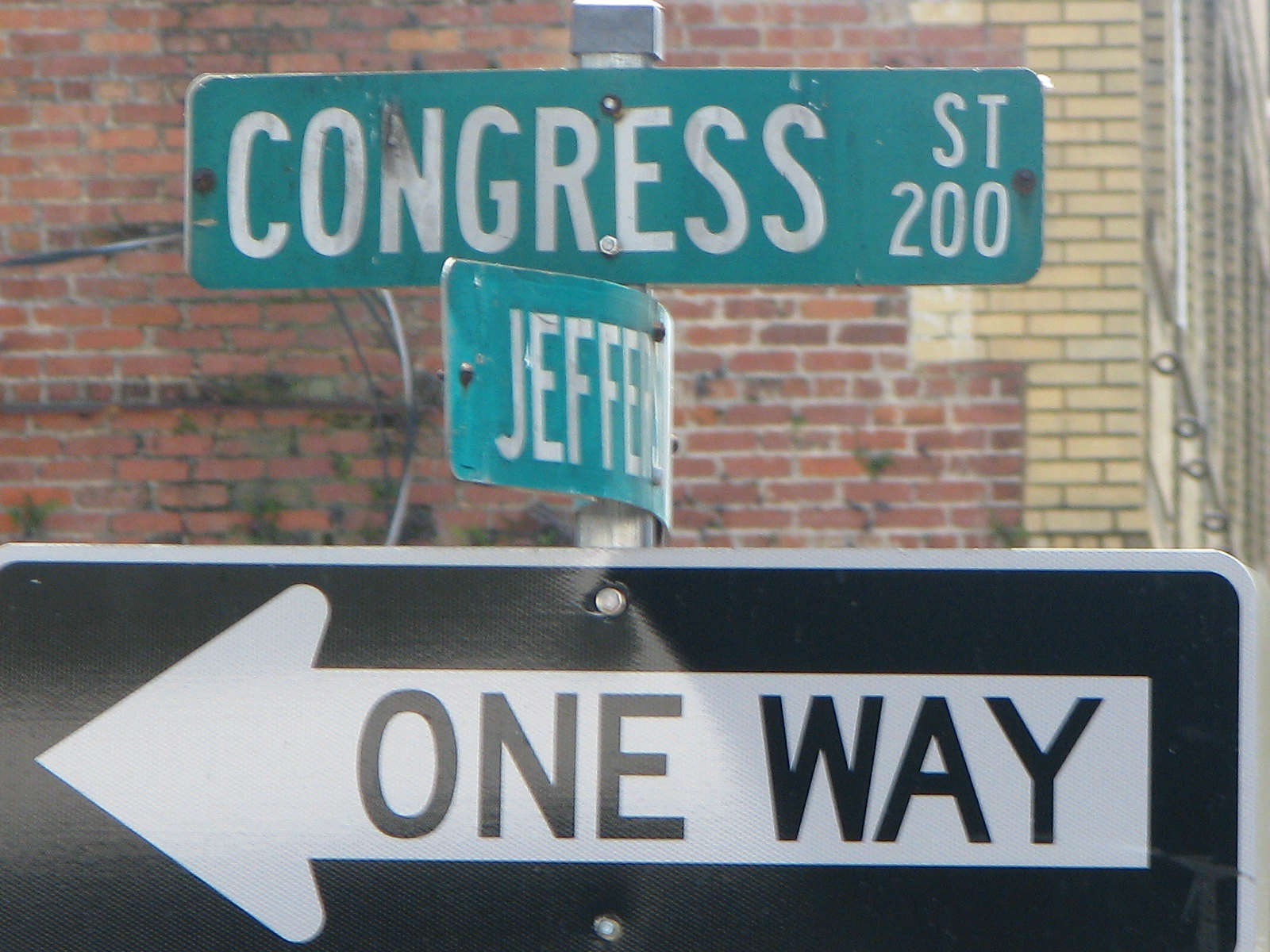In the background, a wall with red bricks interspersed with black shading can be seen, creating a rugged texture. To the right, the wall transitions into a section made of white bricks. Dominating the foreground stands a metal pole capped at the top. Attached to the pole is a green street sign with white text reading "CONGRESS" in the main field. Above "CONGRESS," in smaller text, "STREET" is inscribed to the top right, and below it, the number "200" is listed. The pole features two visible bolts securing the sign in place. 

Lower on the pole, a slightly tilted green sign contains the word "Jeffrey," but the rest of the text is obscured. At the bottom of the pole resides a black square one-way street sign, with a white arrow pointing left and black text alongside the arrow stating "ONE-WAY." The middle street sign appears to be bent, creating a visually uneven display.